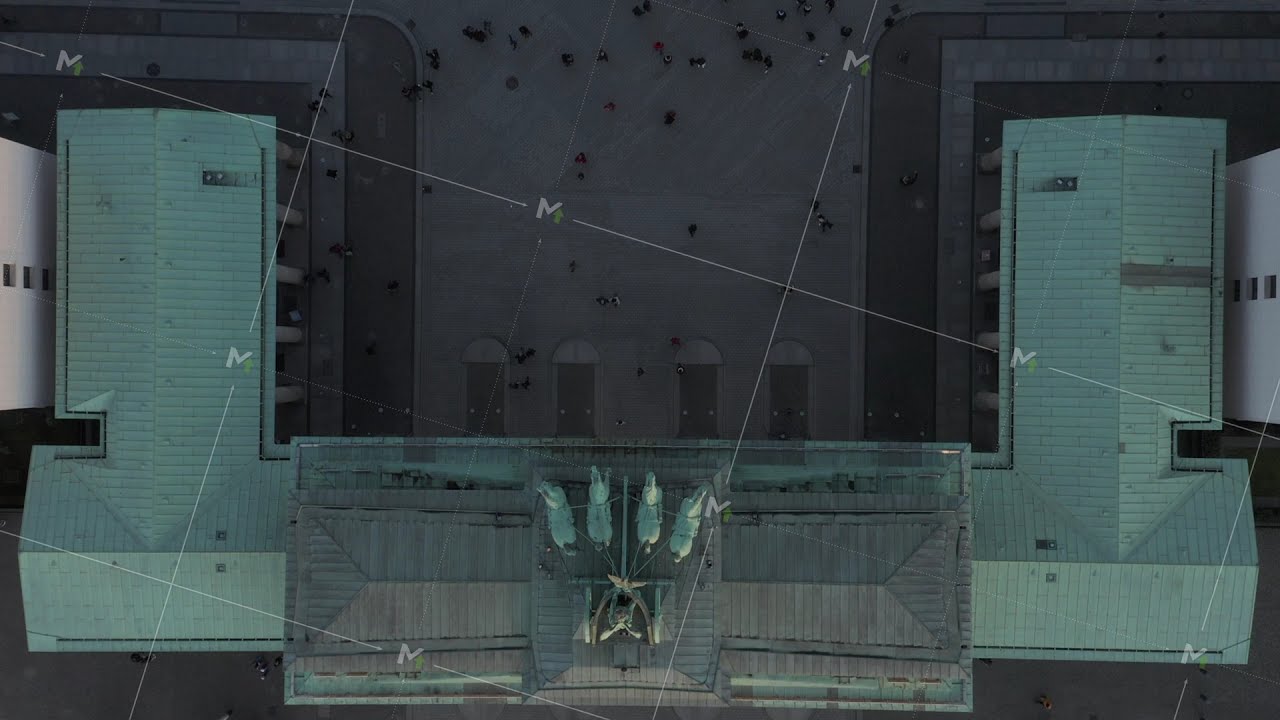The image depicts a top-down view of a uniquely designed building. The building's layout consists of a wide main strip running horizontally near the bottom of the image, with two perpendicular extensions jutting out from each end, forming a broad U-shape. The building’s light green roof, reminiscent of oxidized metal, features a central section with sloped sides and a distinct gray strip that is elevated above the rest. This central strip is adorned with sculptures, including a chariot being pulled by four horses. The camera captures the scene from an elevation of about 60 feet, offering a clear view of the intricate decorations and structure. Within the U-shape created by the building's extensions, there is a courtyard populated with people milling about, giving the area a lively atmosphere.